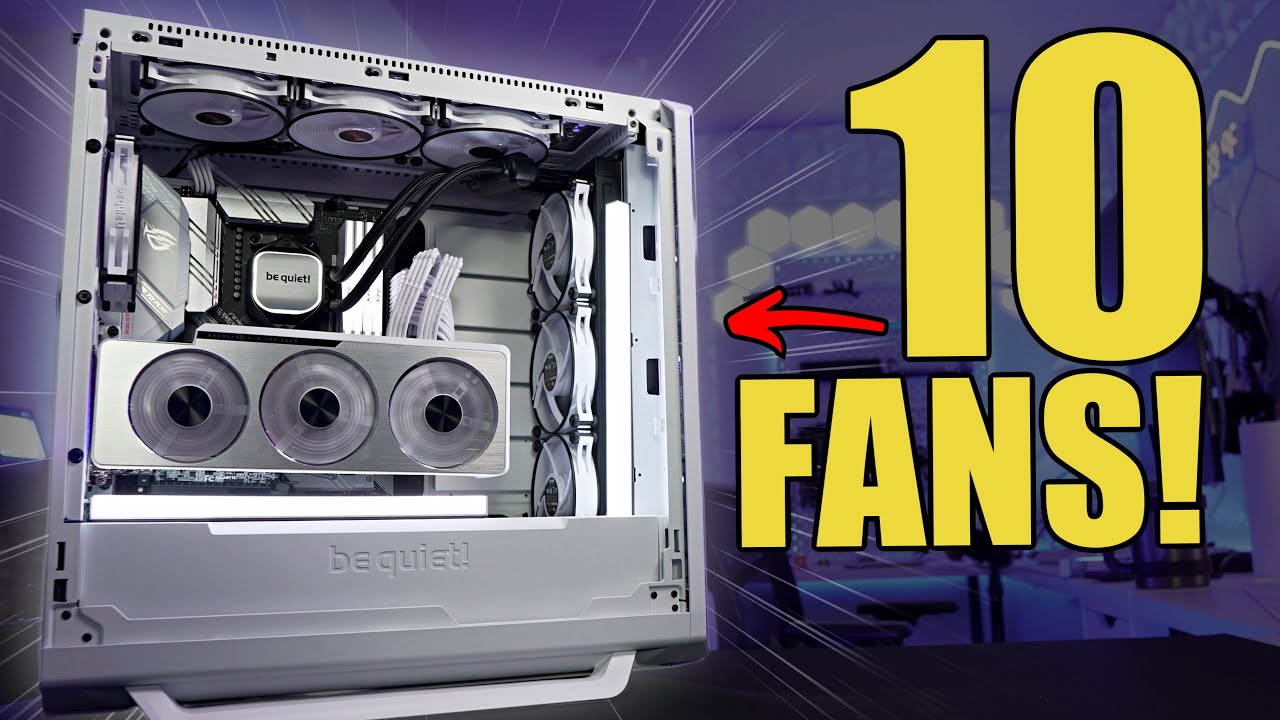The image shows the interior of a high-performance gaming PC tower with its side panel removed, offering an unobstructed view of the meticulously organized components inside. Prominently displayed in large, bold yellow text on the right side of the image is the phrase "10 fans," indicated by a red arrow pointing towards the open tower. Within the case, there are indeed nine visible fans arranged in three assemblies, each consisting of three fans strategically placed to optimize airflow throughout the system. These assemblies are positioned at various locations within the case, contributing to efficient cooling of the high-end components.

The tower itself is branded with the name "be quiet," signifying either the model or manufacturer known for producing noise-reducing computer hardware. This branding appears clearly on a square component inside the tower, and is inscribed again on a part near where the side panel usually attaches. Despite the dense array of fans and cables, the internal layout remains tidy, showcasing black cords neatly channeled through plastic strips that manage the wiring.

In the background, the image features some less discernible elements and spotlights, which slightly obscure additional details but add depth to the presentation. Overall, the caption conveys the complexity and precision engineering of this state-of-the-art gaming rig, emphasizing its cooling capabilities and quiet operation.